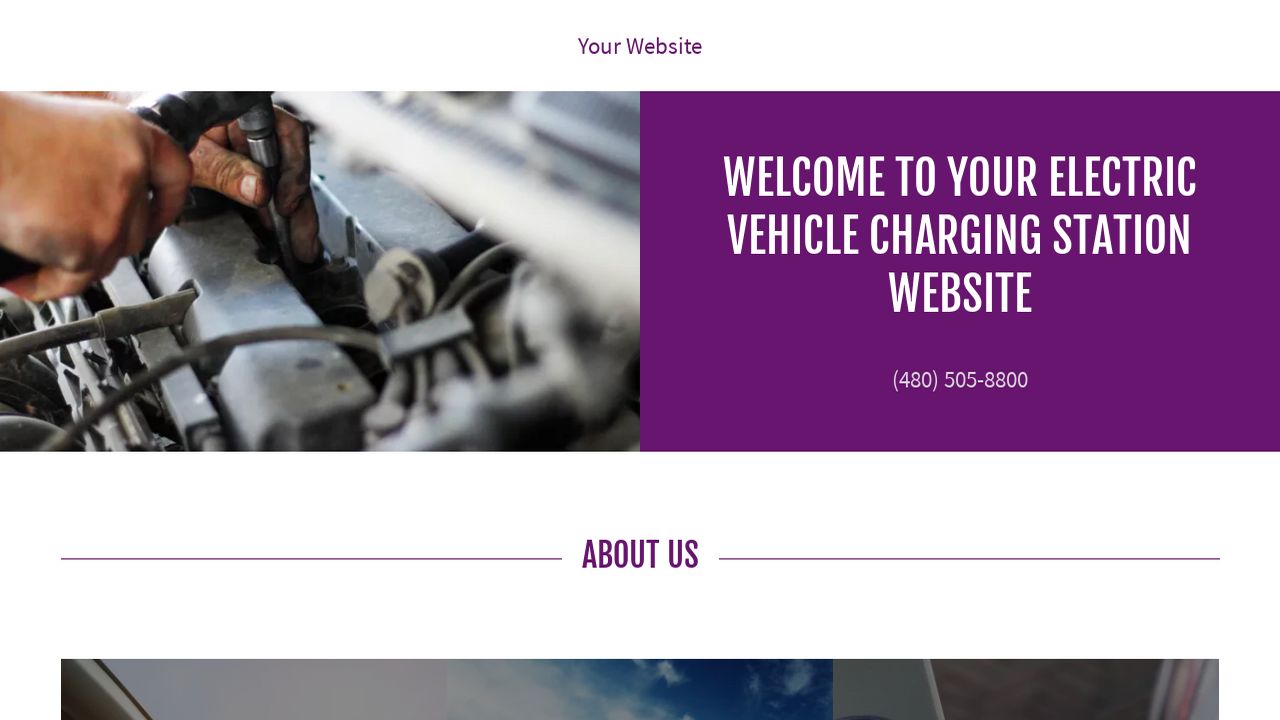The image is a screenshot, likely captured from a laptop or desktop computer, given the dimensions. It appears to be from a website specializing in electric vehicle charging stations. At the top, there is a header that reads "Your Website," potentially indicating that this is a sample website created by a web design platform like Shopify. 

On the left side of the screenshot, there is an image of a mechanic working on a car. The mechanic has oil-stained hands and is using a wrench to work on the vehicle. To the right of this image, there is a purple background with white text that reads, "Welcome to Your Electric Vehicle Charging Station Website." Below this text is a faintly visible phone number: 480-505-8800. Separating these sections is a line with the label "About Us." Beneath this section, there is another image, but it has been cropped out and is not fully visible. The overall background of the website is white, and there are no additional descriptions provided.